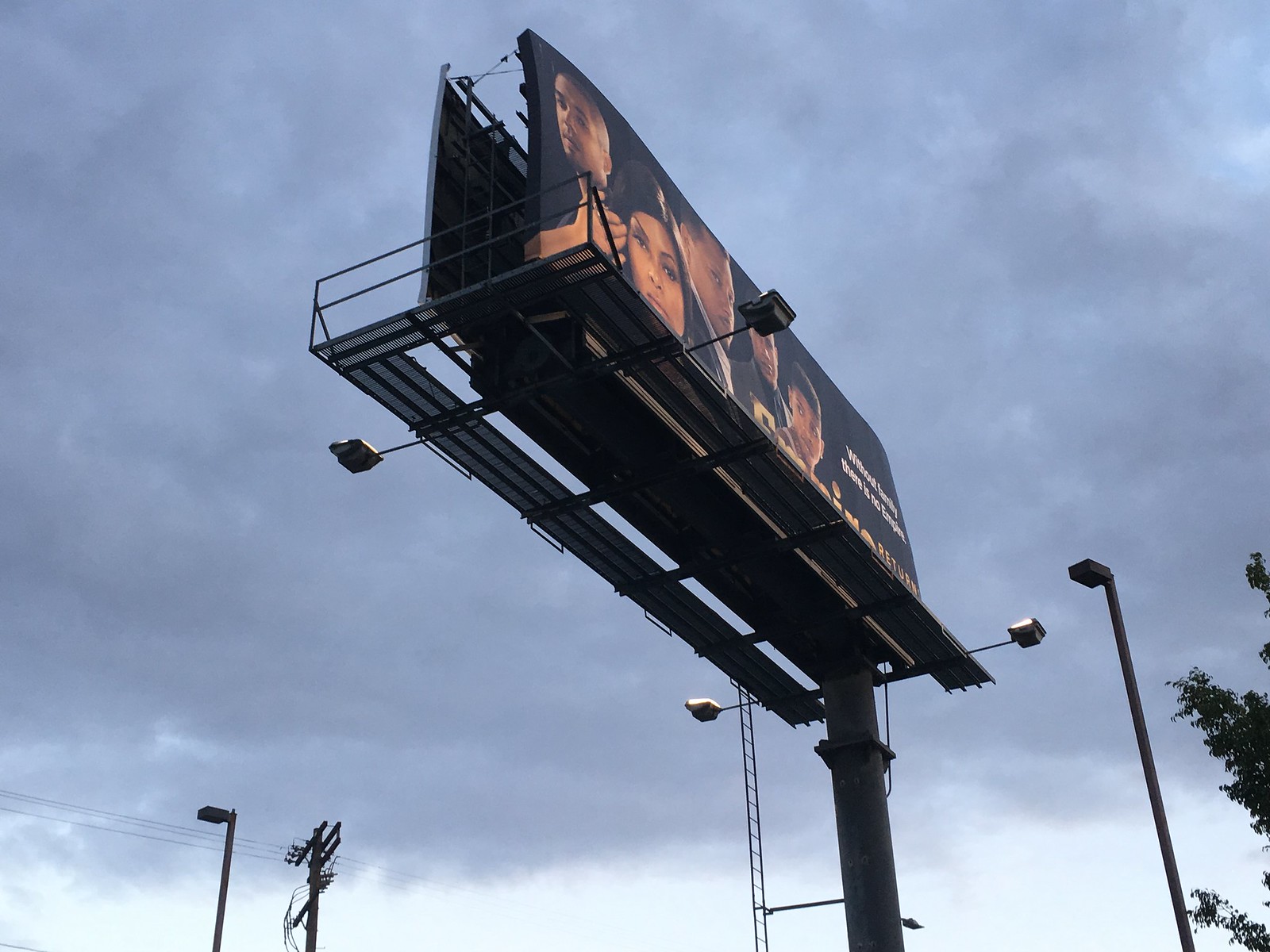This is an overcast, daytime photograph captured from a low angle, looking up at a large billboard outside. The dark gray and blue storm clouds above hint at an impending storm, contrasting with the grayish-blue, overcast sky, creating a moody backdrop. The billboard advertises the television show "Empire," as indicated by the partially visible white text at the top right corner that reads "Empire Return." It features five dark-skinned characters, including the prominent face of Taraji P. Henson. All characters have black hair and are displayed against a black background, with some wearing black shirts. One male character on the right wears a black shirt with a golden letter or number. Another character, dressed in a black shirt with a white undershirt, also has black hair. The individual at the back left sports a brown buzz cut and dons a black shirt. Supporting the billboard is a large cylindrical pole and surrounding it are features such as a dark gray or black scaffolding walkway for maintenance, black-framed lights with white illumination, and unlit square street lights on tall poles. The right side of the photo also contains a dark green tree, adding a natural element to the urban setting.